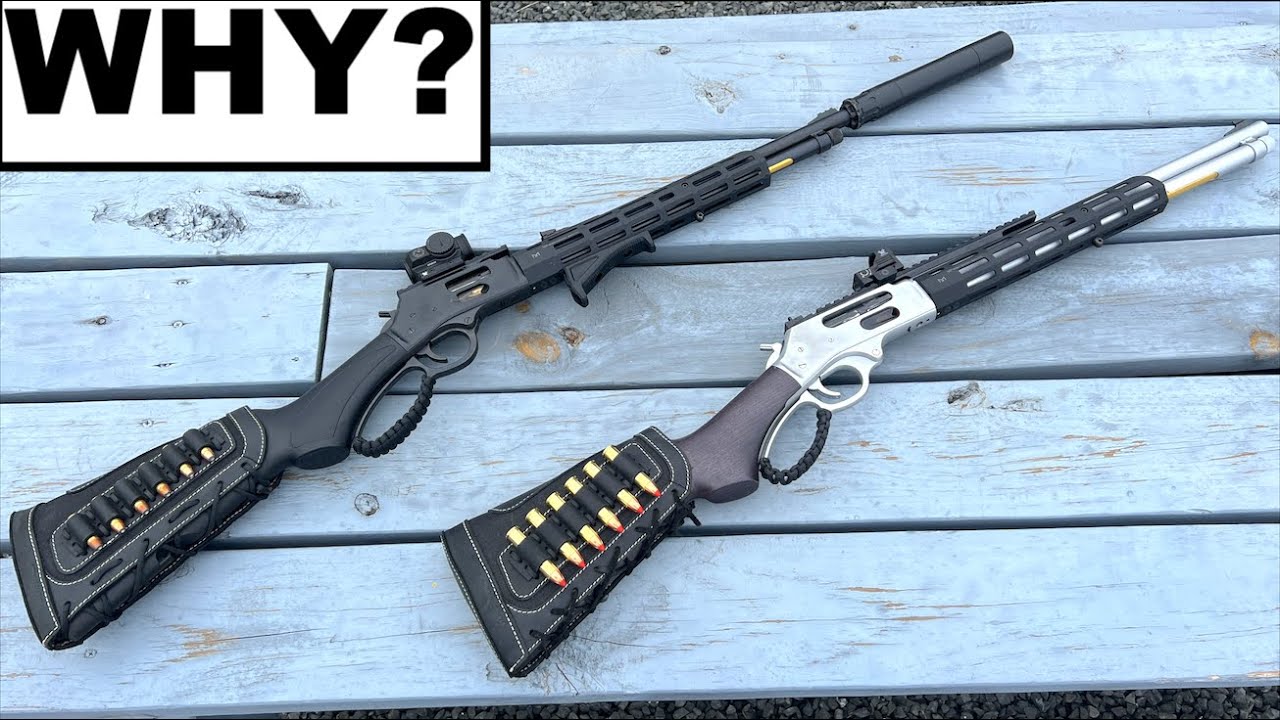A photograph depicts two specialized bolt-action lever-action rifles displayed on what appears to be a wooden benchtop with a grayish or bluish tint. The benchtop planks run horizontally, and the rifles are laid parallel to each other at approximately a 45-degree angle to the wood. There is text in black letters in the top left corner that reads "WHY?" 

One of the rifles is entirely black, featuring a suppressor and a small sighting scope. It has a saddle that holds bullets attached to the butt end of the gun. The second rifle is predominantly black with silver accents and lacks a suppressor. Instead, it has a modern gripping mechanism at the front and a removable sight along the top. A similar holster-like apparatus for holding bullets is attached to its butt end. The setting appears to be an outdoor area, possibly a gravel parking lot, as indicated by some background elements resembling a picnic table.